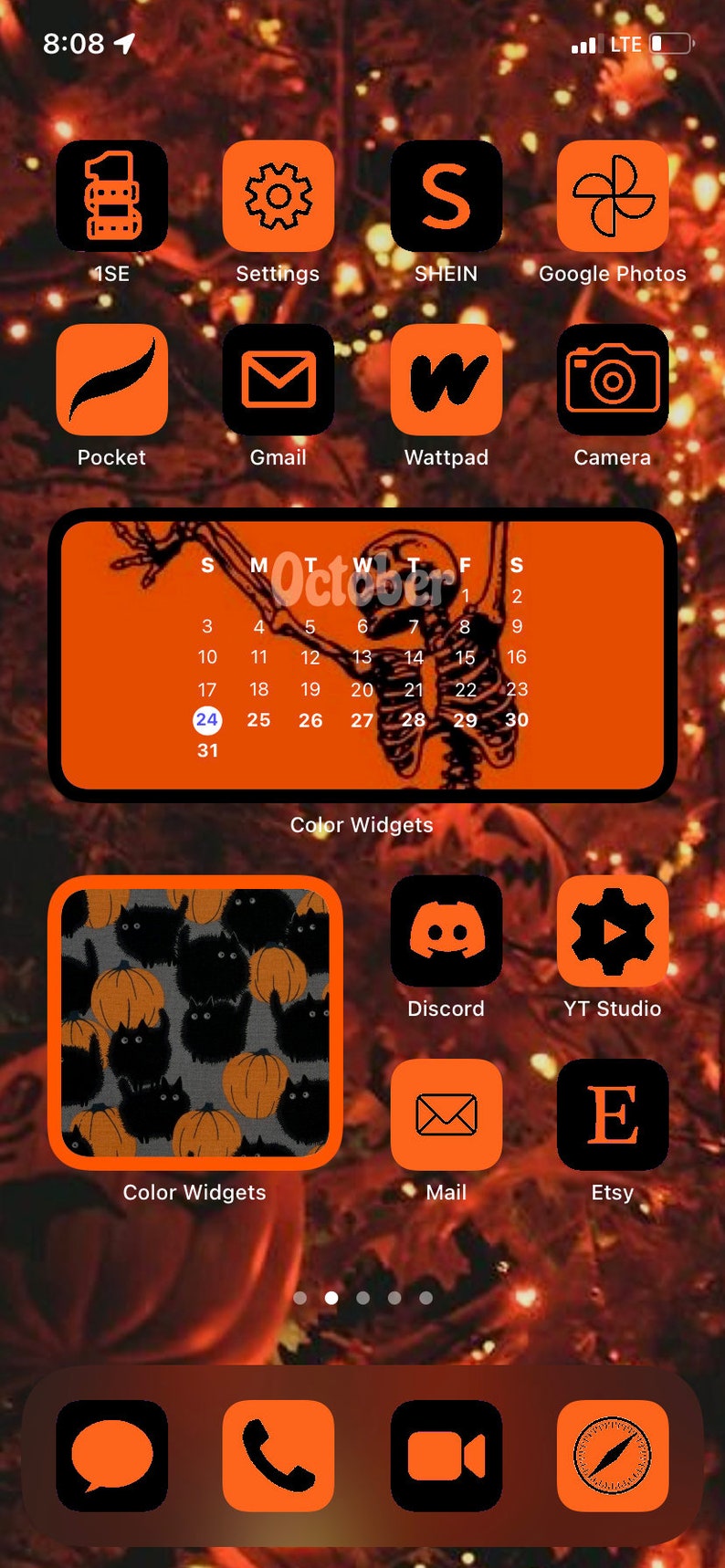This image is a screenshot of a cell phone home screen, captured during the Halloween season. The background is festively decorated with a fall theme, featuring orange lights, pumpkins, and scattered orange leaves that evoke the ambiance of Halloween. In the upper left corner of the screen, white text displays the time as 8:08. The upper right corner indicates the connectivity status with 3 out of 4 bars for LTE signal strength.

All the app icons on the screen have been customized with a Halloween aesthetic, predominantly using shades of orange. In the top left position, there is an icon labeled "S1SE." Directly next to it is the Settings app, reimagined in an orange box. Following that are the Sheen and Google Photos apps, also set against orange backgrounds. The Pocket app is similarly themed, followed by Gmail, which is displayed as a black box with an orange envelope. Other noticeable apps include Watchpad and the camera app.

Prominently displayed beneath these icons is the current month, October, encapsulated in an orange rectangle. Adjacent to the month is a graphic illustration featuring half of a skeleton from the waist up, enhancing the spooky Halloween theme.

On the lower left side of the screen, there's a large rectangular bordered box. This box is adorned with cute illustrations of kittens and pumpkins, adding a whimsical touch to the otherwise spookily themed home screen.